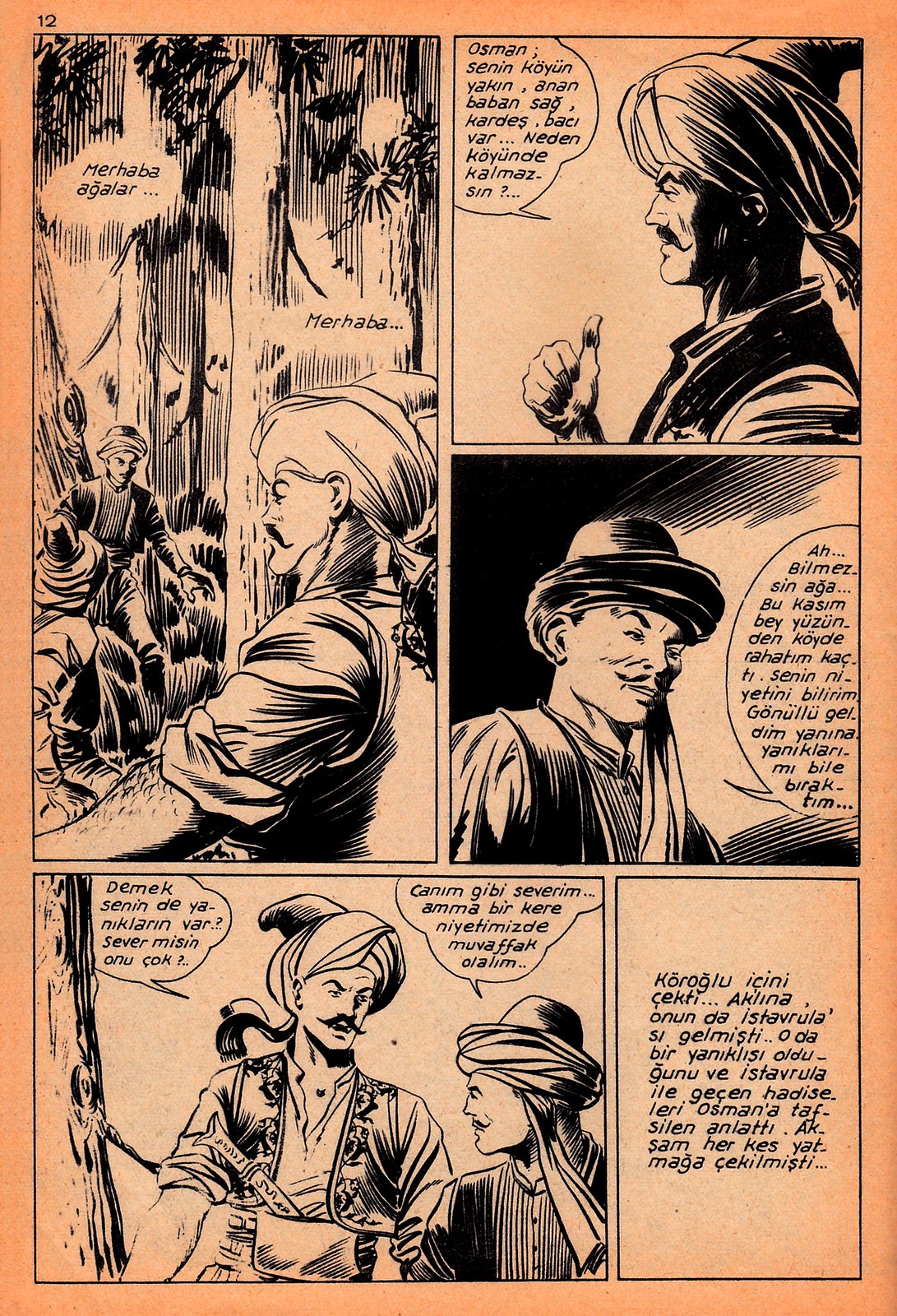The image showcases a sepia-toned comic book strip consisting of five detailed panels, rendered with professional, high-quality artwork. In the top-left corner, the strip features text in a foreign language. The central figures are two male characters, both adorned in traditional attire: long-sleeved robes and turbans, hinting at a setting possibly in Persia or South Asia. One of the men is depicted with a mustache and a vest, giving a thumbs-up in a serious demeanor, while the other, similarly mustached, appears equally solemn in his billowy shirt and vest. The fourth panel sees these two characters standing by a tree, seemingly in conversation, their expressions and the presence of speech bubbles adding to the narrative. The entire composition, though primarily in sepia, exudes a rich, illustrative quality, further emphasized by the intricate detailing and professional finish of the drawings.